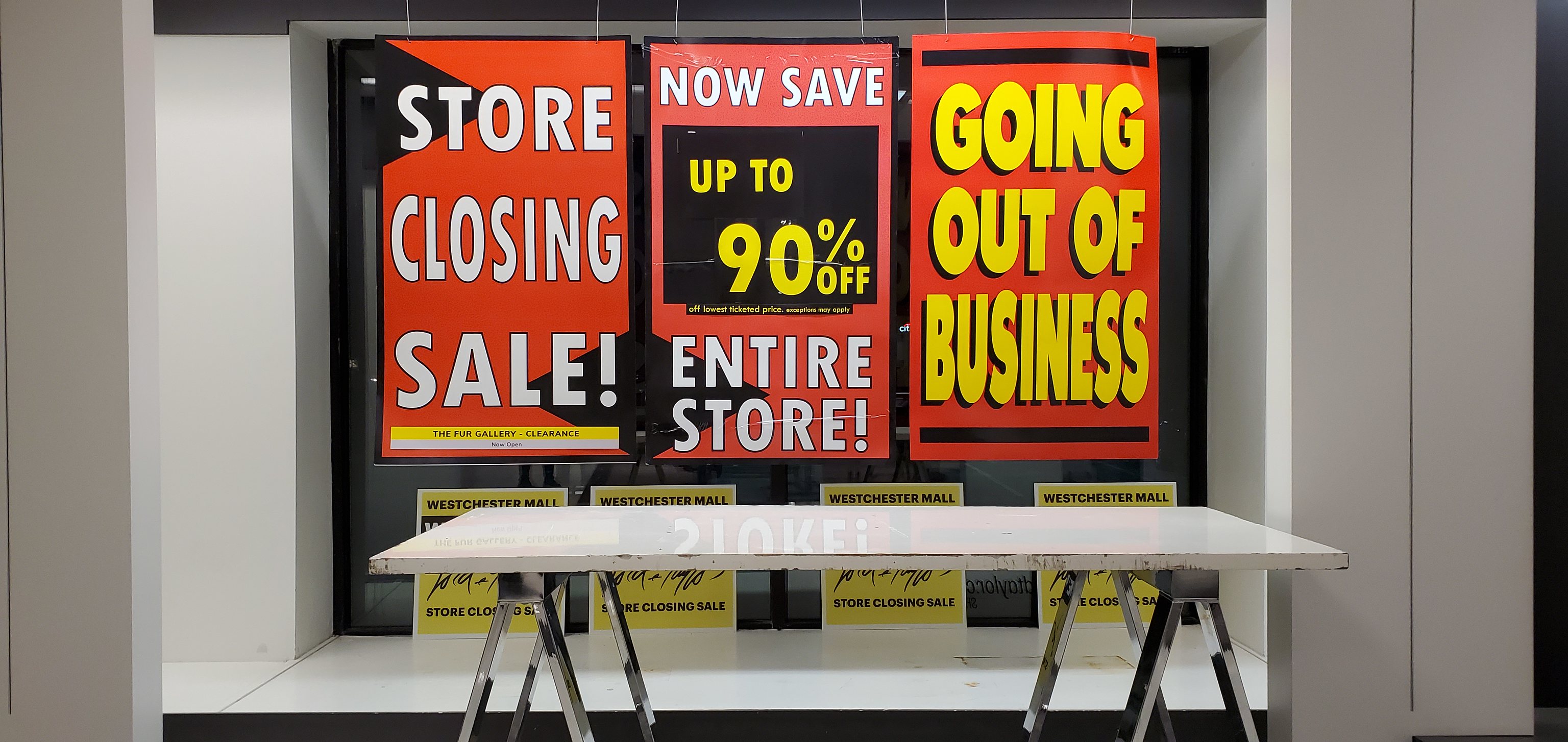This sharp photograph captures a storefront at Westchester Mall, prominently featuring three large red signs with white and yellow text. The sign on the left announces, "Store Closing Sale!" Below it, a smaller sign reads, "Fergallery Clearance, Now Open." The central sign declares, "Now Save Up To 90% Off, Off Lowest Ticketed Price, Exceptions May Apply, Entire Store!" while the sign on the right states simply, "Going Out Of Business." Along the bottom of the storefront, four identical signs are propped up but partially obscured by a white work table in front. Despite the obstruction, the visible text reads "Westchester Mall" and "Store Closing Sale." This image vividly captures the urgency and finality of a major retail sale event.